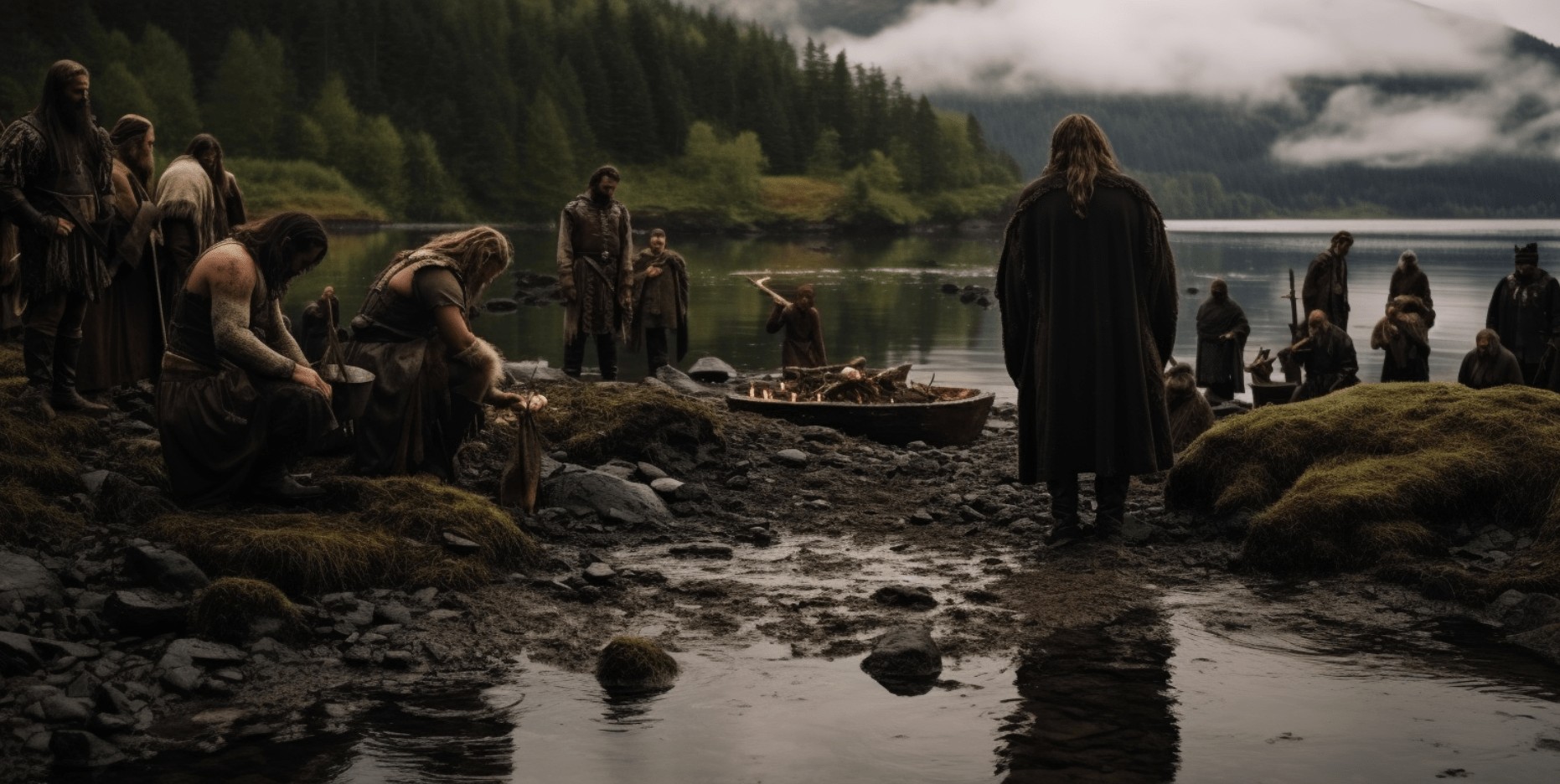The image is a rather dark, rectangular photograph that evokes a somber atmosphere. Dominated by hues of dark green, olive green, dark brown, and a touch of tan, it captures a cloudy, shadowed scene that might be at dawn or dusk. The primary focus is a small boat, similar to an oar-powered vessel, beached on a slender sandbar that bridges two rocky landmasses—the left enclosed by a thick tree line and the right framed by more rocks and a forested background. 

A group of about 20 men, all appearing as dark, indistinct figures, populates the scene. On the left bank, five men are visible; three stand while two kneel or squat, seemingly engrossed in looking down, possibly at tools or weapons. Standing at the heart of the sandbar is a large man in a long, dark overcoat, notable for his obscured features. To his left and closer to the boat are three men, two looking downward, perhaps paying attention to something on the sand or the boat itself, which might carry candles.

On the right side of the boat, six to eight men stand, partially veiled by the dim light. The overcast sky, heavy with gray and white clouds, casts a dreary pall over the scene, making the entire tableau appear as a still from a shadowy, atmospheric movie.